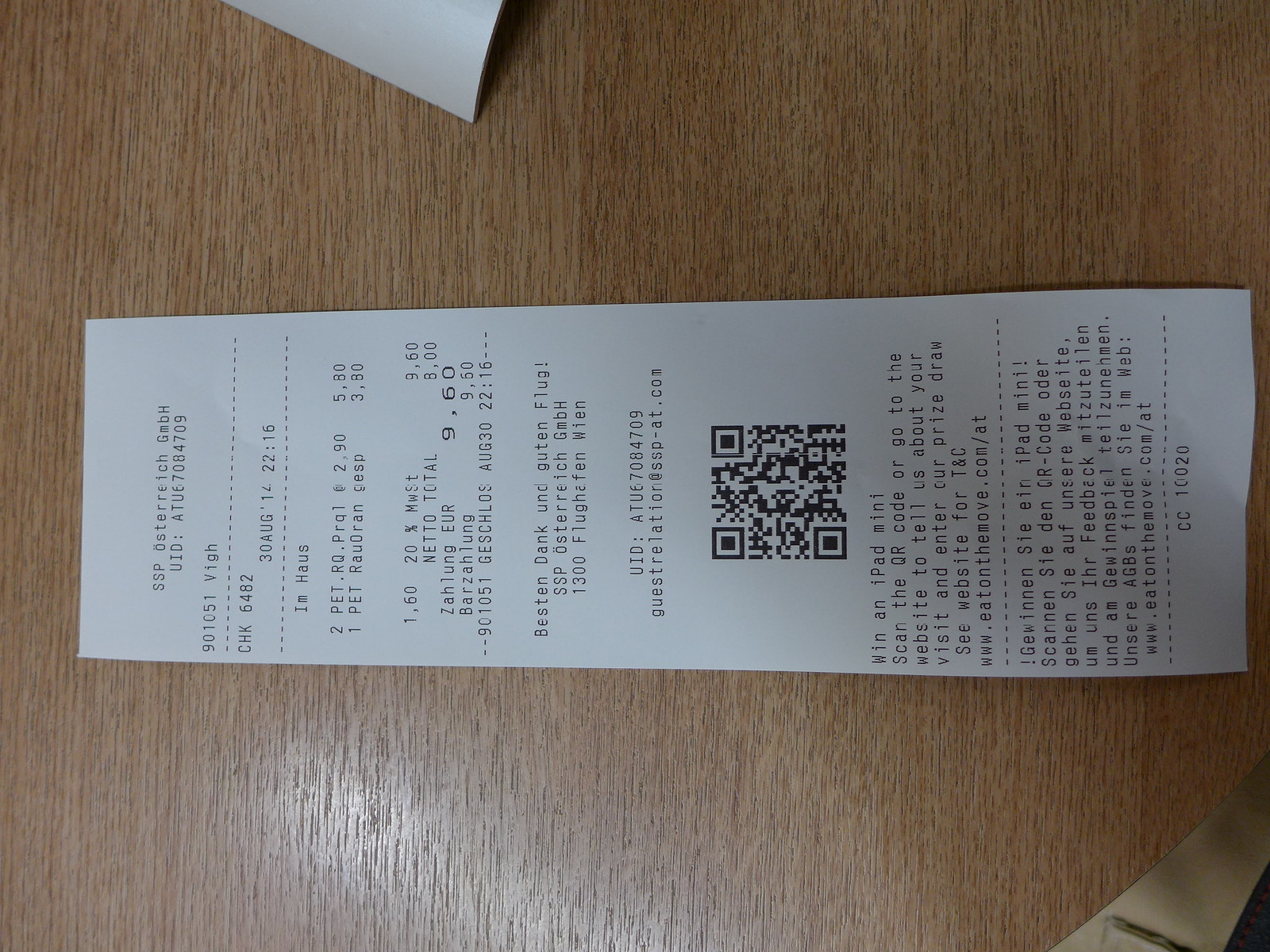The image captures a thermally printed paper receipt, laid sideways with the top of the receipt positioned to the left, on a brown woodgrain table with the grain running vertically. The receipt, from SSP Osterreich GmbH, is printed in German and documents the purchase of two items totaling €9.60. A QR code is prominent just right of center, followed by a bilingual message in English and German. The English text invites the customer to "win an iPod mini" by scanning the code or visiting www.eatonthemove.com.at to provide feedback and enter a prize draw. Details on the receipt include phrases like "Bestendank und Guten Flügel" and the retailer's name, SSP Osterreich GmbH.